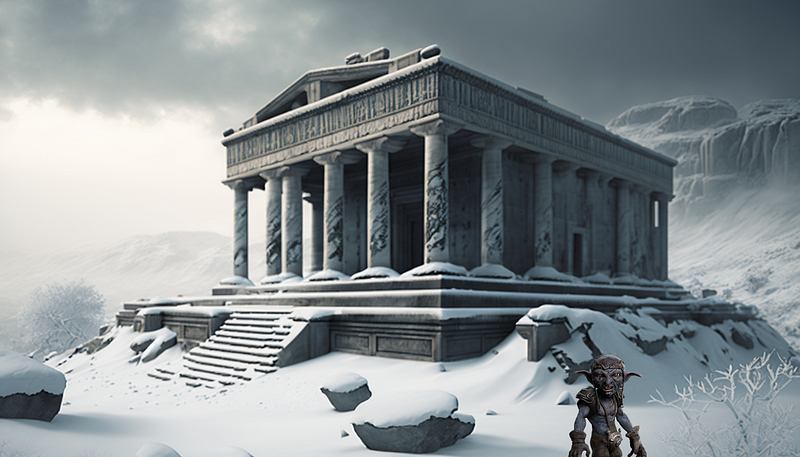In this detailed fantasy image, an animated or computer-generated scene unfolds under a cloudy, overcast sky that hints at a dusky environment. Dominating the foreground is a small goblin-like creature with an oversized head, pointy ears that curve outward, grayish skin, and yellow eyes. The goblin, donned in minimal attire that includes a headgear, gloves, shoulder pieces, pants, and a water flask, stands to the front right, facing slightly toward the back.

The backdrop of the scene features a desolate, snowy landscape with scattered, dark gray, snow-covered rocks and boulders. At the very center rises an imposing, Parthenon-inspired structure, reminiscent of Greek or Roman architecture. This marble building appears abandoned, characterized by its numerous pillars—six at the front and six along the sides—massive steps leading to a recessed doorway, and a weathered appearance that adds to the ancient and forlorn atmosphere.

Beyond this stately edifice, a mountain range stretches into the background, their snow-clad peaks almost blending seamlessly into the gray, cloud-filled sky, which further deepens the sense of isolation and timelessness of this frozen tableau.